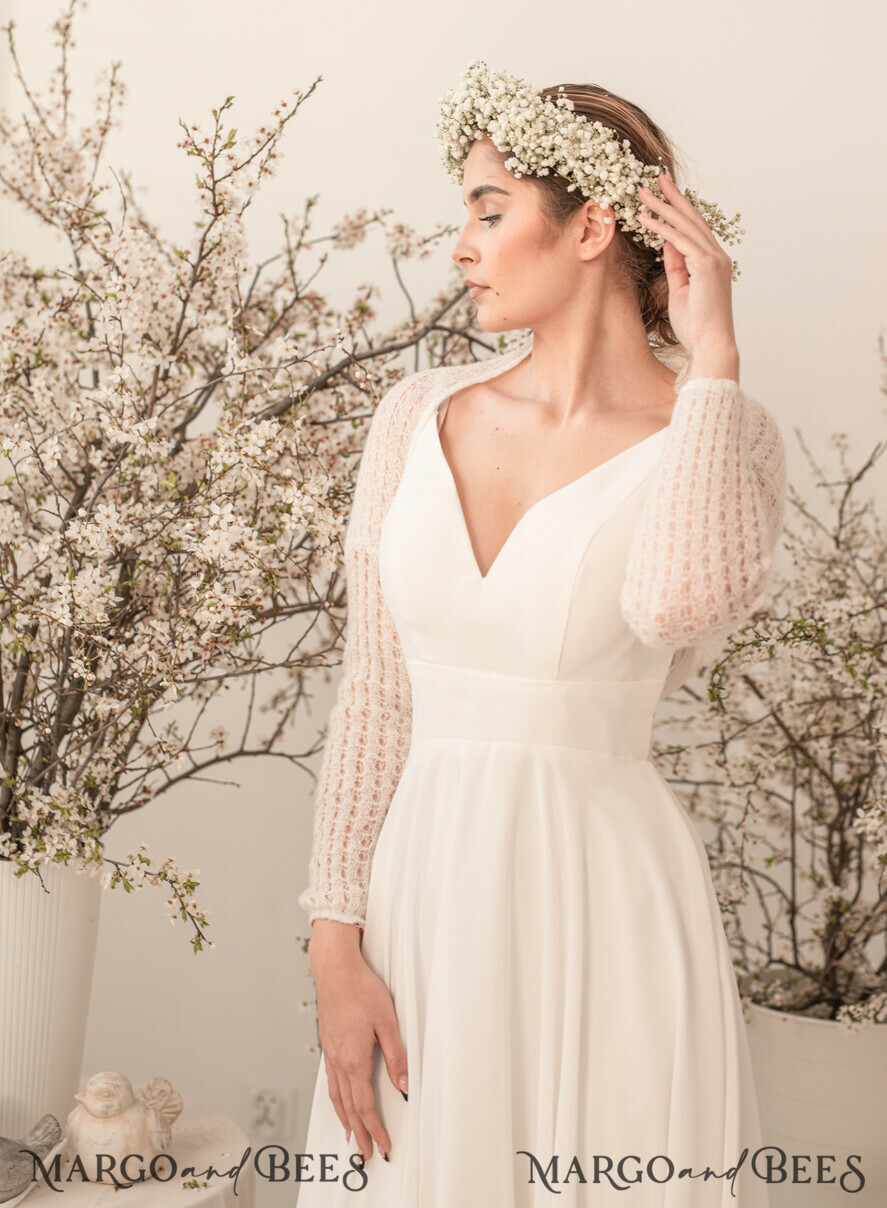In this captivating advertisement by Margot and Bees, a woman in her 20s or 30s elegantly models an ethereal ensemble. She is dressed in an ivory V-neck dress with a plunging front and lacy, sheer long sleeves that reveal a glimpse of her skin underneath. Her nails are meticulously manicured with black tips, adding a modern twist to her timeless look. Adorning her head is a delicate wreath of small white flowers, akin to what a flower girl might wear, which she gently holds with one hand while the other hand rests gracefully on her thigh. She gazes thoughtfully to the left, her brown hair tied back and makeup flawlessly applied. The serene setting features a white wall complemented by white vases and pots filled with branches of tiny white flowers, reminiscent of forsythia but in white bloom. A charming statue of a dove sits beside one of the pots, adding to the tranquil ambiance. The watermark "Margot and Bees" is elegantly inscribed in a feminine script at the bottom of the image.